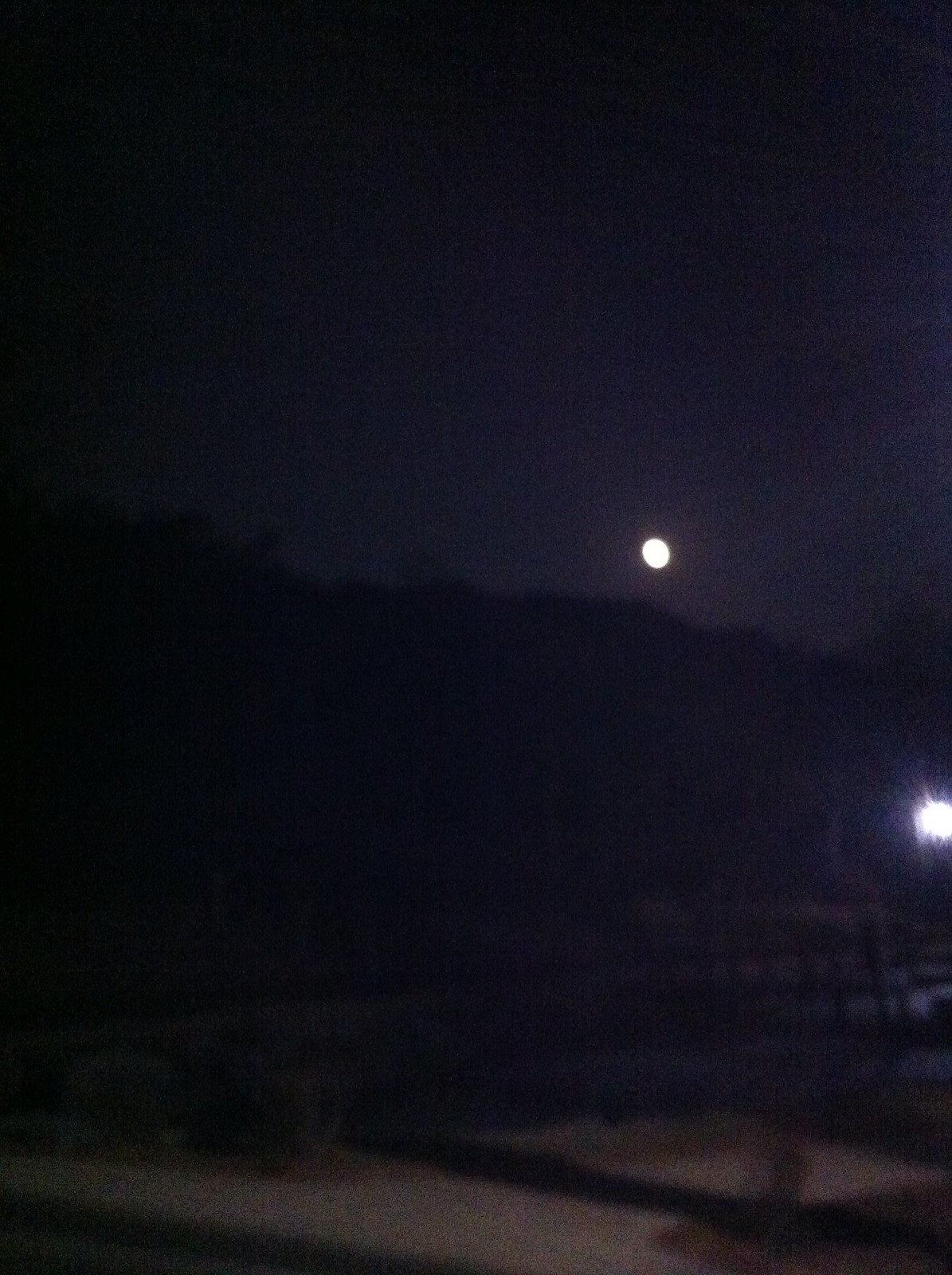In the nighttime photograph, the moon, roughly three-quarters full and glowing a yellowish hue, takes center stage in a clear, dark sky devoid of stars. Positioned off-center, it hovers above the faint, black silhouette of a distant hill. Just below the center-right of the image, a bright, white light, presumably a construction or night lamp, illuminates the scene, casting a stark contrast with its intense luminosity. This light source is even more brilliant than the moon due to its proximity and bathes the foreground in a light gray hue. A long, vertical shadow extends from the bottom right, though its origin remains unclear. In the backdrop, subtle shadowy figures likely represent trees or a forested area, adding depth to the scene. Despite the clear sky, the overall image is slightly blurry, lending an indistinct and bland quality to the nightscape.